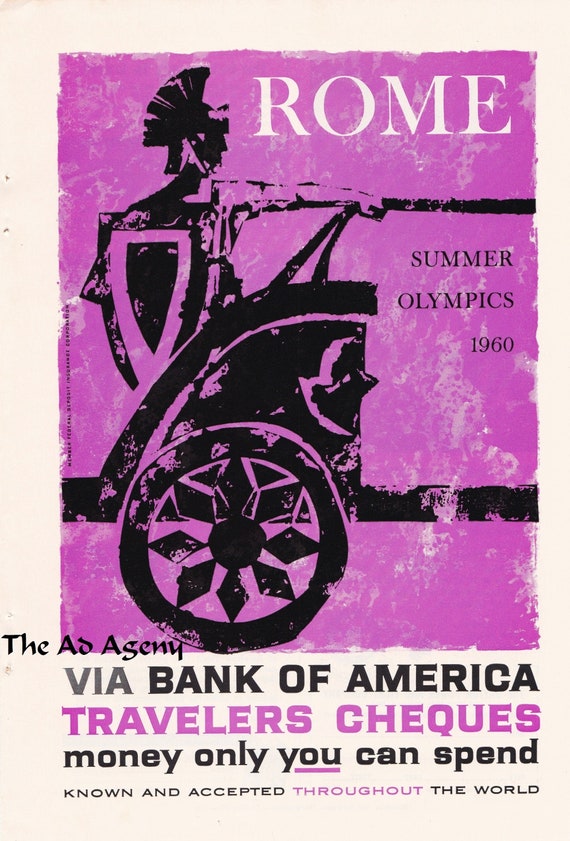This vintage-styled poster advertises the Rome Summer Olympics of 1960. The central image is a lithograph print featuring a Roman soldier in a chariot, rendered in black and white (or perhaps black and purple) against a rough purple background. The Roman soldier, wearing a helmet, holds a shield in one hand and the reins of the chariot in the other. At the top of the image, the word "Rome" is prominently displayed in white print, while directly beneath it, in black print, the text reads "Summer Olympics 1960." The lower section of the image contains an advertisement reading, "The Ad Agency, via Bank of America Traveler’s Cheques: Money Only You Can Spend, Known and Accepted Throughout the World." This implies sponsorship by Traveler’s Cheques, emphasizing their global acceptance. The overall composition features a white background framing the purple and black imagery and text.